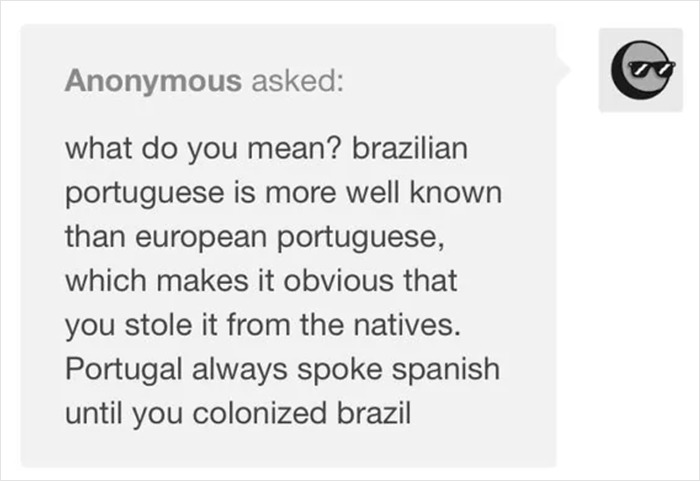This image is a cropped screenshot from a social media platform, highlighting a unique chat interface. The chat bubble is unconventional in its design, being square instead of the typical round shape. Positioned to the right is the profile picture—an anonymous grey square icon featuring a circle with sunglasses as a simplistic face representation. On the left side is the comment box, which dominates the majority of the white space. The comment box itself is grey and is bordered by a thin, almost imperceptible, light grey line, defining its rectangular shape.

At the top of the comment box, there's a header in bold dark grey font that reads "anonymous asked." Below this header, the message content is displayed: "What do you mean? Brazilian Portuguese is more well known than European Portuguese which makes it obvious that you stole it from the natives. Portugal always spoke Spanish until you colonized Brazil." The entire layout underscores the anonymous nature of the interaction while focusing attention on the controversial comment.